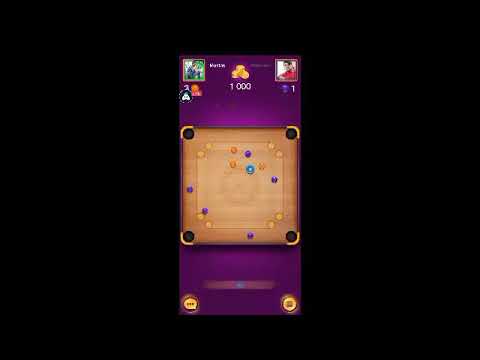The screenshot depicts a smartphone game set against a solid black background, with a thick black border forming a frame around the image. The game screen features a tan-colored square resembling a wooden board with small, colorful dots—blue and orange—scattered across it, akin to marbles. The board's corners have black holes, evoking a pool table's pockets. A prominent royal purple border is at the top and bottom of the screen. The top center showcases a stack of gold coins with the number "1000" in white beneath them.

In the top left and top right corners are tiny, indistinct profile pictures, which are likely real photos but too small and blurry to discern specific details. The bottom left corner contains a gold-colored speech bubble icon with three black dots inside, representing a chat feature. The bottom right corner features a gold circle with a smaller brown rectangle, the exact function of which is unclear but likely serves as another interactive element in the game.